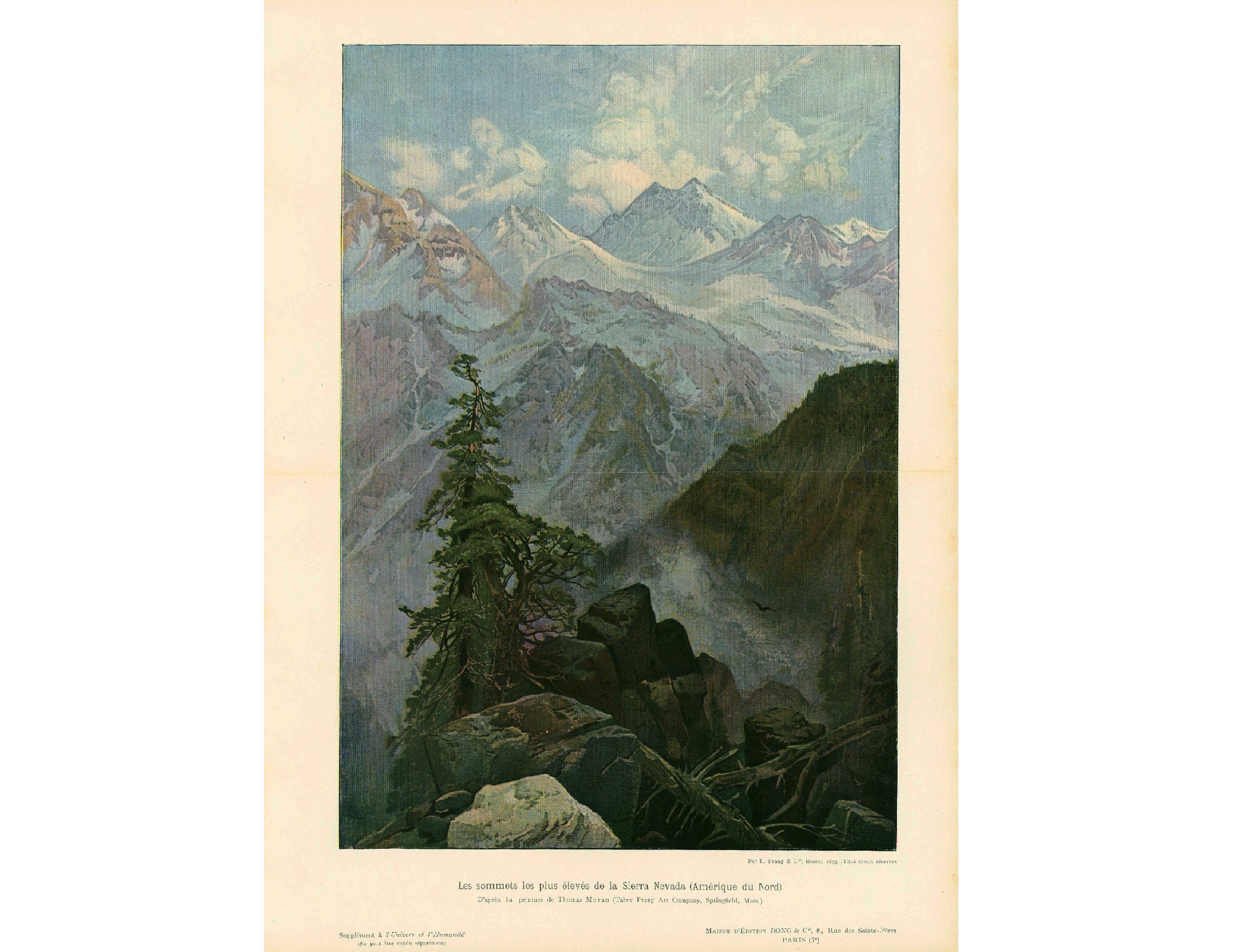The image is a detailed landscape painting of a mountainous region, printed on an off-white postcard that creates a border around the central picture. Dominating the foreground is a dark brown rocky outcropping, atop which grows a singular, large green pine tree. This rugged outcrop is accented by surrounding boulders and rocks. Midway through the composition, a forest-like area with possibly evergreen trees flows into the scene, leading the eye toward larger hills and, subsequently, a backdrop of towering snow-capped mountain ranges. The nearest mountains have patches of brown visible beneath a light layer of snow, whereas the distant peaks are almost entirely enveloped in white, stark against the sky. A wisp of steam or smoke can be seen near the front, to the right of the primary tree. The painting, which exhibits qualities reminiscent of an oil painting or tapestry, features a caption below it in black font, possibly in French, identifying the name of the painting, the artist, and the date of creation. The postcard captures this scene with rich detail, evoking the grandeur and serene beauty of the natural landscape.